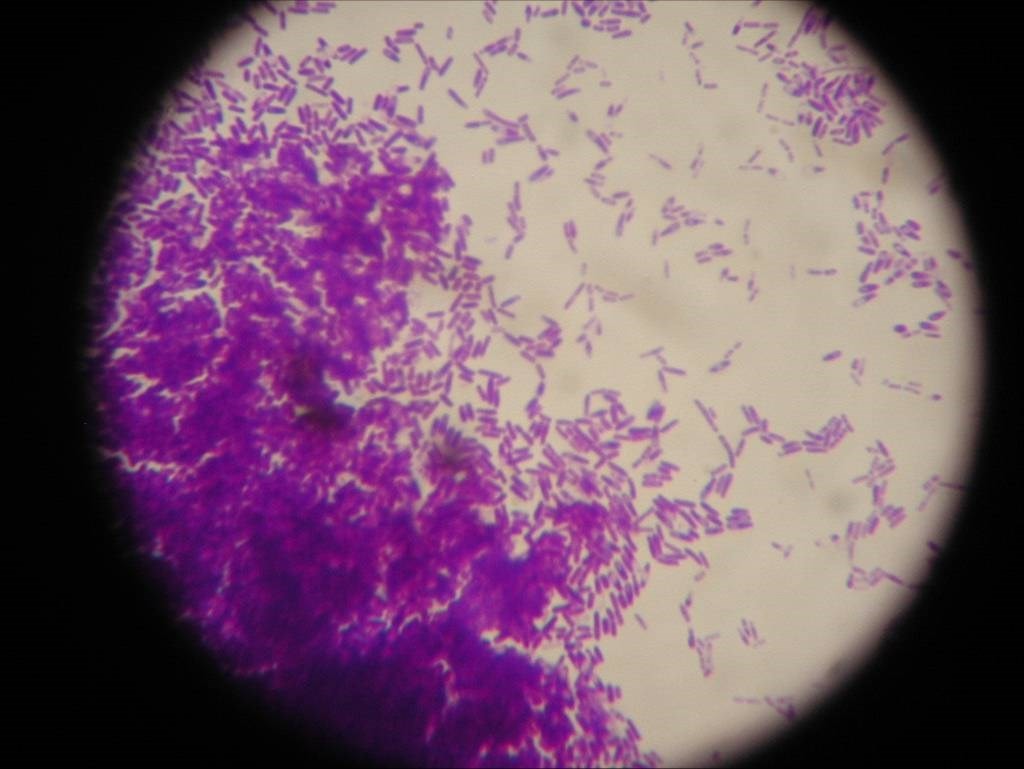The image depicts a black rectangular background featuring a prominent circular disk in the center that resembles a microscopic slide view. The disk shows a beige or light tan background with sporadic darker spots. A notable feature within the disk is the presence of numerous purple areas. The darkest and most concentrated of these purple masses are predominantly located on the lower left side of the circle, where they form a dense, dark border along the rim. As they extend out from this area towards the upper right, the purple specks become progressively lighter and more dispersed. These purple areas vary in form, with some appearing as interconnected clumps while others are free-standing. The visual effect suggests the specks might be tubular-shaped bacteria cells or similar microscopic entities.